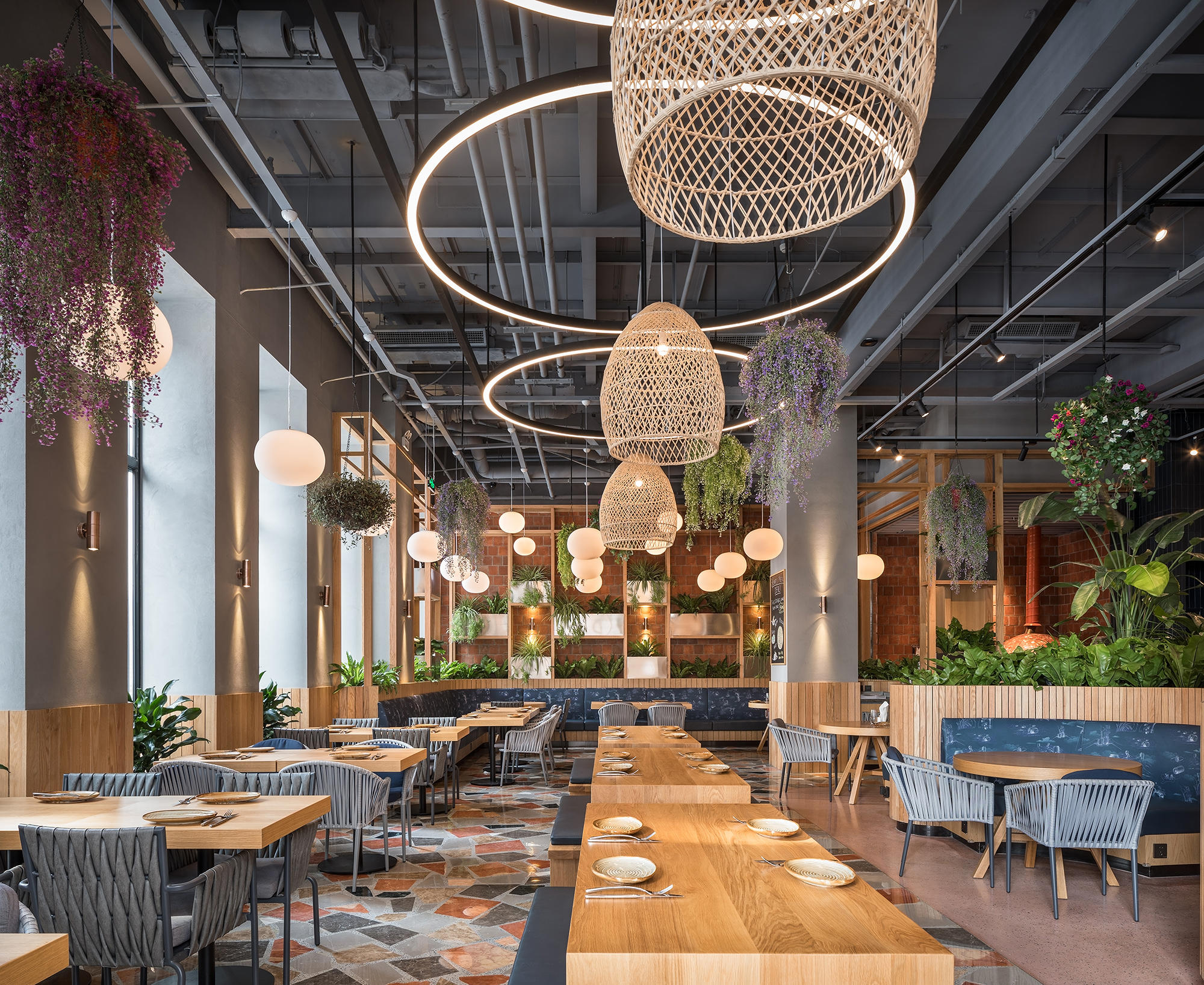The interior of this modern, beautifully designed restaurant features a spacious layout with a variety of seating options and an abundance of greenery. At the center are three long wooden tables set for four, each adorned with white plates and silverware, surrounded by gray chairs. Flanking these tables are smaller, classic wooden tables, each also set for four, but with dark plates and silverware. The seating includes cushioned bench seats in dark blue with white accents and additional circular tables and booths that provide a cozy dining experience.

Above, the ceiling is open and industrial, painted gray, showcasing exposed pipes, ducting, and track lighting. This is complemented by an array of lighting fixtures, including upside-down woven basket chandeliers, LED lights, and bubble lamps, providing a warm and inviting atmosphere. The flooring is a colorful mosaic of gray, dark gray, light gray, and peachish-orange tiles, adding to the eclectic aesthetic of the space.

To the right of the photo, a large pot of greenery with small trees and plants adds a refreshing touch, while the far end of the room features a bar with additional seating. The back wall is adorned with a large garden wall set against exposed brick, and shelves of varying heights also containing plants, contributing to the lush, green theme throughout the restaurant.